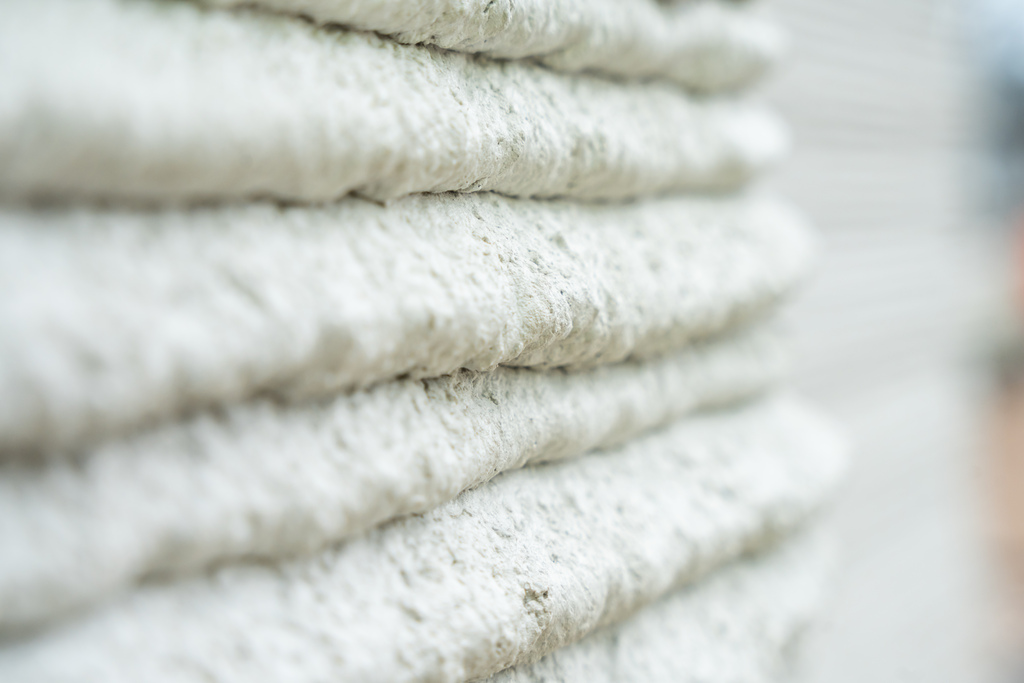This photograph captures a neatly arranged stack of roughly six to seven towels with a textured, somewhat scratchy surface, appearing in a mix of cream and white hues. The towels, layered one on top of the other with slightly rounded edges, are positioned towards the left side of the image, where the focus is sharpest. Both the left and right sides of the frame are blurred, contributing to an unclear background with hints of white, black, and brown tones. The overall orientation of the image is landscape, emphasizing the central stack of towels against the indistinct surroundings.